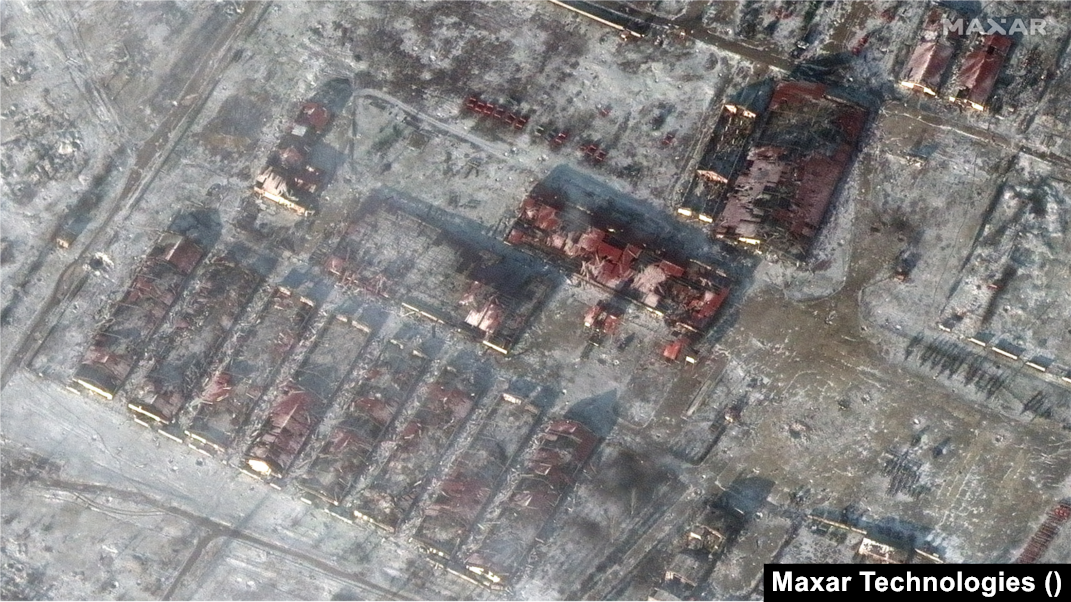This aerial view captures a devastated town, potentially affected by wartime actions. The scene is dominated by rows of closely packed rectangular buildings, most of which have red roofs. Some structures appear heavily damaged or collapsed, their roofs either destroyed or caved in, suggesting significant destruction. The land is predominantly gray, either covered in ash or a light dusting of snow, adding to the desolate atmosphere. Among the destruction, there are larger buildings centrally located and signs of undisturbed areas with parked vehicles, contradicting total devastation. The image, taken during the day, shows the entire area blanketed in a grayish-brown dirt or ash, reinforcing the somber tone. Notably, the bottom right corner features the text "Maxar Technologies," identifying the image's source.